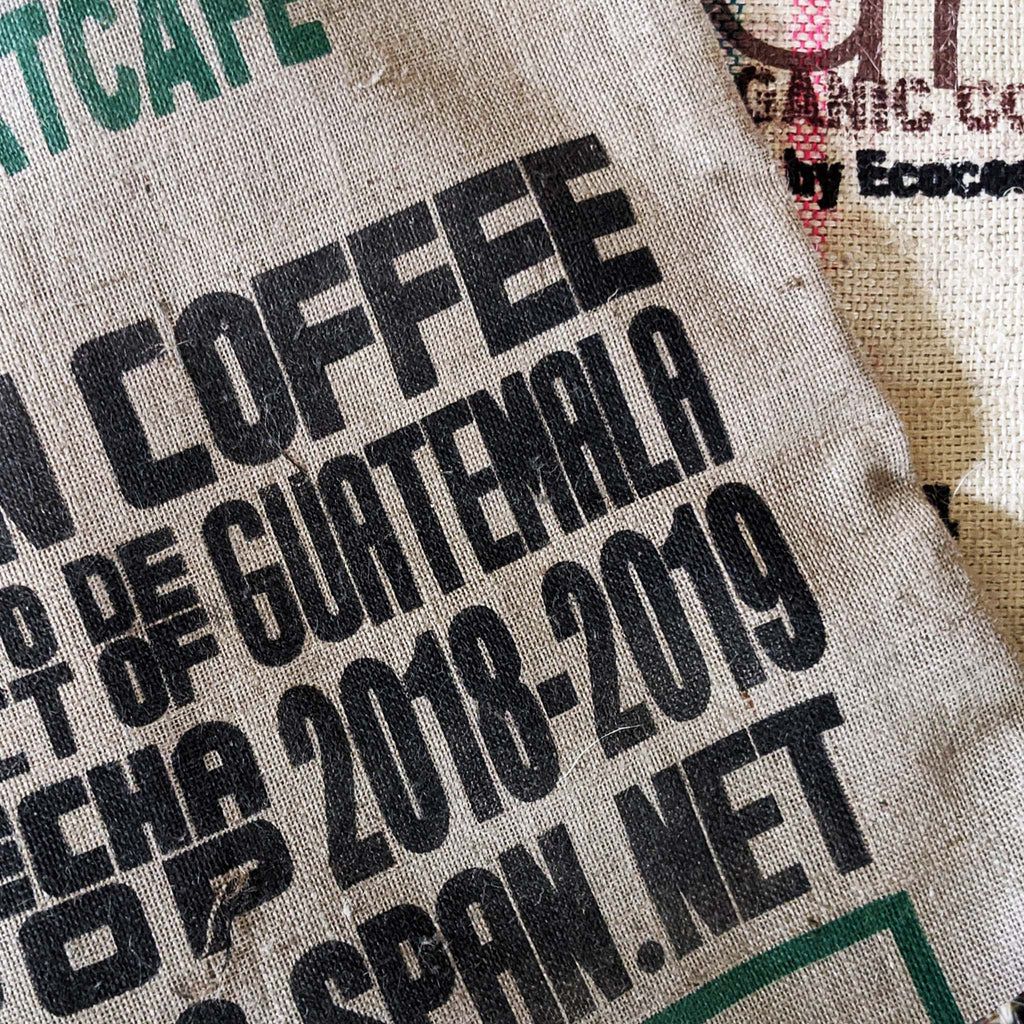The photograph showcases a set of empty burlap coffee sacks. The top sack, in a darker brown hue, prominently features green and black printed text. The green text includes partially visible words and designs, with "cafe" being discernible. The black text reads "COFFEE," "GUATEMALA," "2018-2019," and "SPAN.NET." Additional black text is visible but partially obscured, suggesting something like "ECOCON." The print is in a boxy font. Beneath the top sack lies an off-white sack, with less visible but distinct text. The visible letters "G-A-N-I-C C-O" suggest it is labeled "organic coffee" by "ECO-CON." Overall, the bags are detailed with bold typography and branding elements, indicating their purpose for transporting coffee beans from Guatemala.